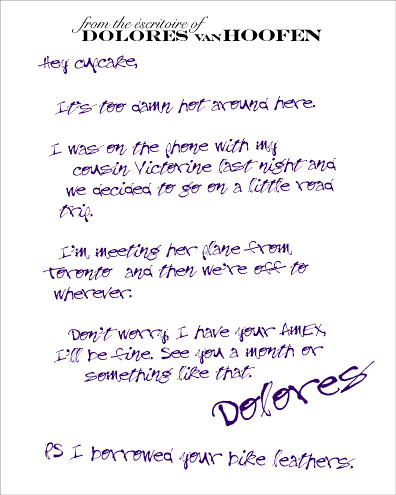This image features a piece of paper with a white background and a very thin in-striped border. At the top, centered in bold black print, it reads, "From the Escritoire of Dolores Van Hoofen." Below that, in whimsical purple handwriting, the note begins, "Hey Cupcake, it's too damn hot around here. I was on the phone with my cousin Victorine last night and we decided to go on a little road trip. I'm meeting her plane from Toronto and then we're off to wherever. Don't worry, I have your Amex. I'll be fine. See you in a month or something like that. Dolores." At a diagonal from the lower left to the upper right, Dolores signs it, and beneath the signature, it says, "P.S. I borrowed your bike leathers." The only colors used are white for the background, black for the printed words, and purple for the handwritten note.